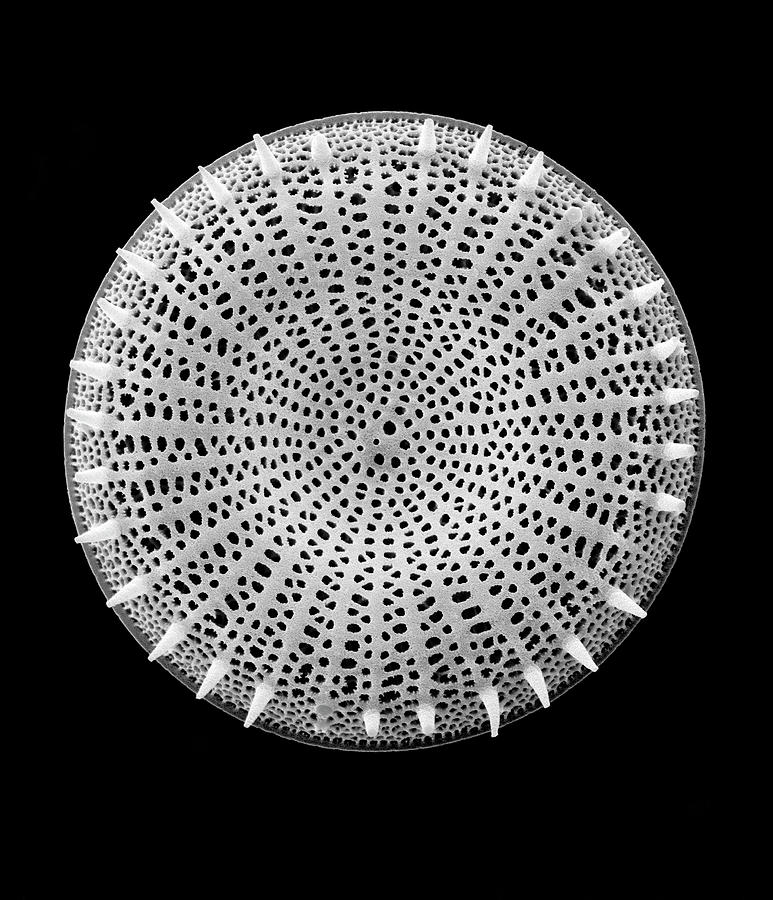The image depicts a computer-generated, metallic silver disc with a pure black background. The disc features an intricate geometric design, resembling something observed under a microscope. Around its edges are numerous white, spiky protrusions forming a circular pattern that spirals outward. The surface of the disc is perforated with numerous uneven black circular holes that extend from the center to the circumference. The center of the disc appears recessed, adding depth to its flat, silver appearance. The combination of spikes and holes gives the object a tooth-like texture that contrasts sharply with the smooth, metallic finish.